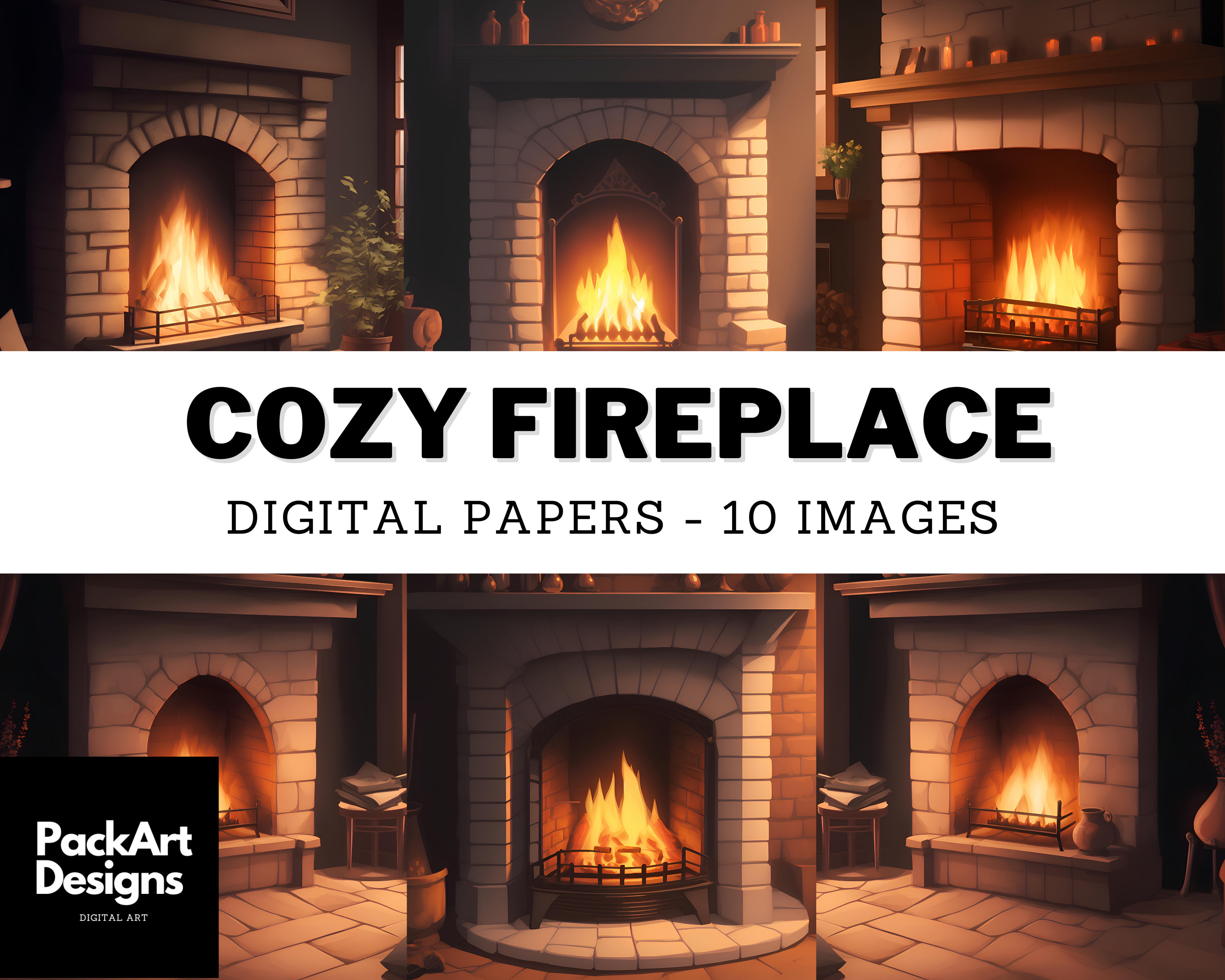The image showcases a visually appealing template or advertisement designed for digital art enthusiasts. At the center of the composition is a prominent white banner with black font text that reads, "Cozy Fireplace, Digital Papers, Ten Images." This banner, resembling a wide horizontal strip, extends across the width of the image from left to right.

Above and below this central banner are rows of three fireplaces each, making a total of six fireplaces depicted in the image. These fireplaces are intricately designed with light gray stone textures and exhibit a cozy ambiance with flames burning inside them, radiating shades of yellow and orange. The realistic appearance suggests the fireplaces are computer-generated digital art.

In the bottom left corner of the image, there is additional text in white font that reads, "Pack Art Designs, Digital Art." This label provides further context about the type of artwork presented.

The overall design is both alluring and practical, effectively combining text and imagery to communicate the concept of a digital paper pack themed around cozy fireplaces.